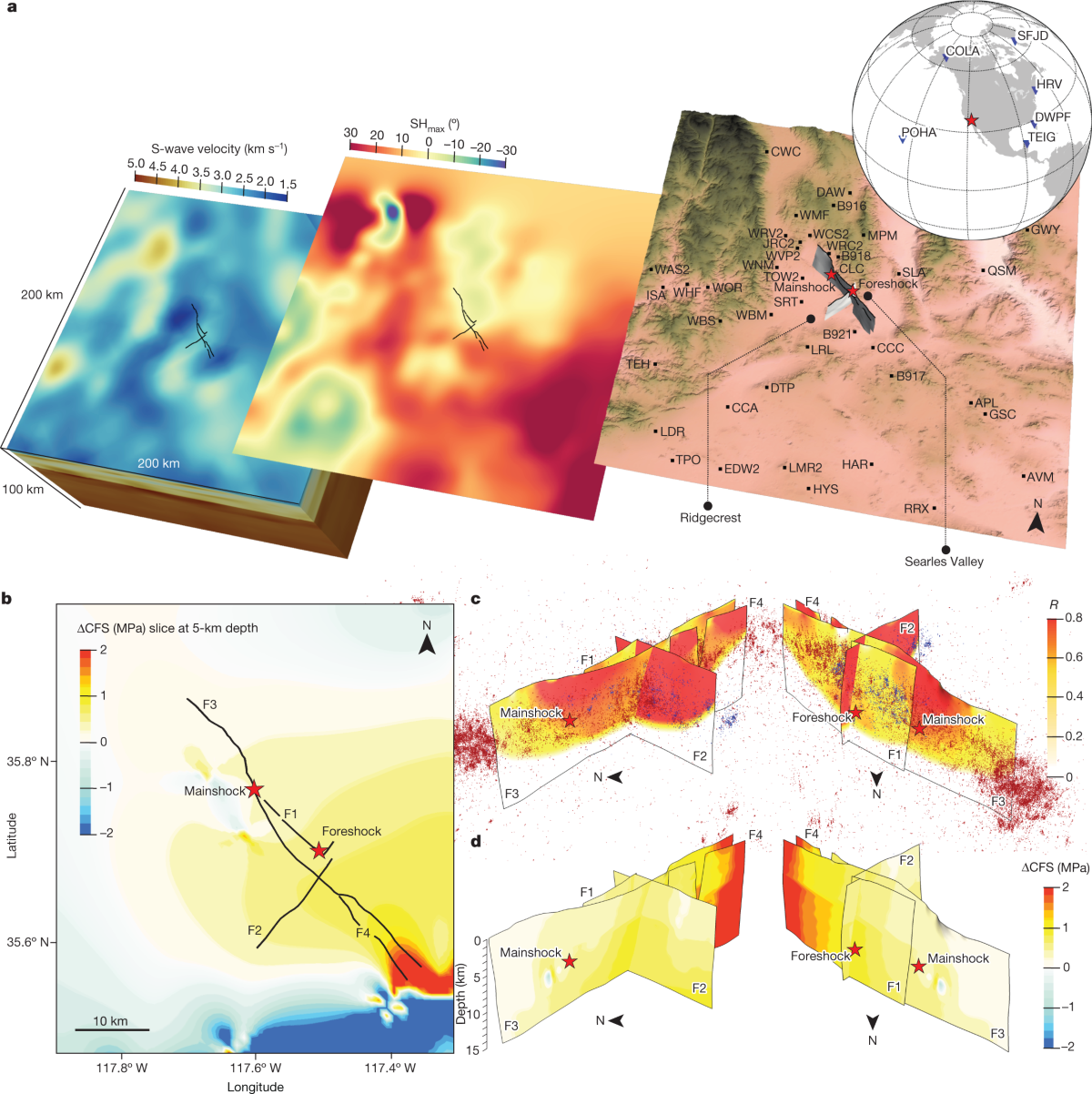The scientific graphic against a white background features a detailed arrangement of maps and radar images depicting S-wave velocity, earthquake intensity, and geographic locations. The top row consists of three diagonally tilted square images. The first square on the left displays a color-coded heat map of S-wave velocity, with a gradient from blue to yellow and a scale ranging from 5.0 to 1.5. The middle square is predominantly red, showing dark red blobs interspersed with patches of orange, yellow, and occasional blue. The rightmost square is a topographical map marked with abbreviations such as WBS, TEH, LDR, and TPL, and includes a contour map with brown and green textures. Above this map is a monochrome globe highlighting locations HRV, DWPV, TIG with blue spots, and a red star near Baja, California.

The bottom row features two vivid radar-like images. The left image shows a gradient of yellow transitioning to orange and deepening to red, with a blue patch at the bottom and a vertical scale ranging from -2 to 2 along the left side. The right image includes scattered red points and additional layered diagrams without red points, likely illustrating earthquake intensity and depth variations. The overall imagery suggests a comprehensive study of seismic activity, with emphasis on geographical mapping and intensity metrics.